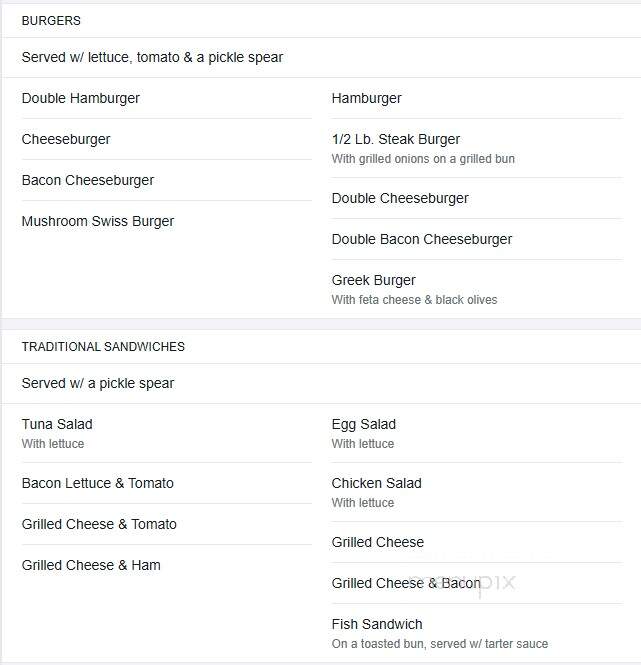**Descriptive Caption:**

A black-and-white portrait-oriented image depicting a computer-generated restaurant menu. The layout mimics a printed paper menu, with no visible interactive features like buttons to select or add items to a cart. The header sections of the menu categorize different meal types distinctly. 

At the top, the "Burgers" section lists a variety of options, all served with lettuce, tomato, and a pickle spear. The choices include:
- Double Hamburger
- Cheeseburger
- Bacon Cheeseburger
- Mushroom Swiss Burger
- Hamburger
- Half Pound Steak Burger
- Double Cheeseburger
- Double Bacon Cheeseburger
- Greek Burger

Below the burgers, the "Traditional Sandwiches" section offers items that are served with a pickle spear. Options here include:
- Tuna Salad
- Bacon, Lettuce, and Tomato (BLT)
- Grilled Cheese and Tomato
- Grilled Cheese and Ham
- Egg Salad with Lettuce
- Chicken Salad with Lettuce
- Grilled Cheese
- Grilled Cheese and Bacon
- Fish Sandwich (served on a toasted bun with tartar sauce)

The design's minimalist color scheme features a white background with all text printed in black ink, accentuating the straightforward presentation of the menu items.